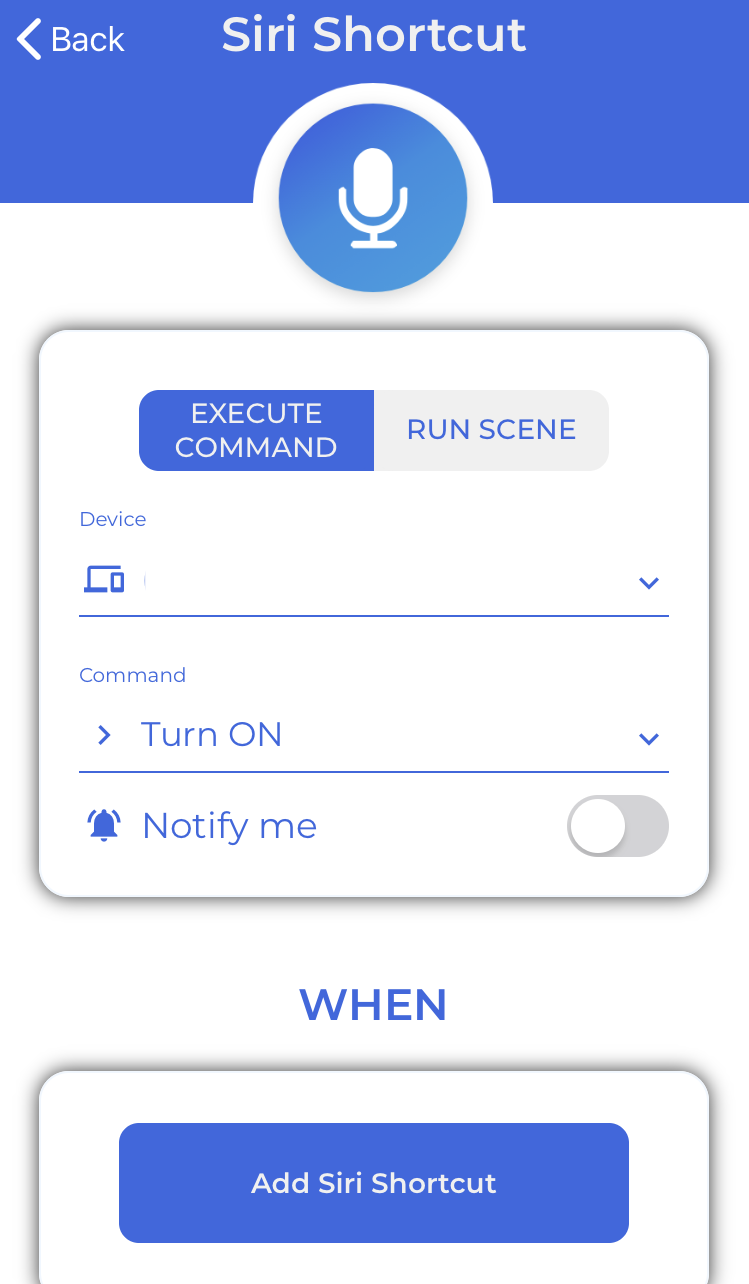This is a detailed screenshot of a Siri Shortcut page. At the top of the page, there is a blue bar that spans across the entire screen. On the left side of this blue bar, there is a back button represented by a white arrow pointing left and labeled "Back" in white text. Centered within the blue bar, the text "Siri Shortcut" is prominently displayed. Below this blue bar, slightly cutting into it, sits a circular blue microphone button.

The main section of the page starts with a white rectangular box titled "Execute Command" at the top. Within this box, on the left side, there is an option labeled "Run Scene" with adjacent blue and gray buttons configured for setting specific commands. Below this, there is a drop-down menu labeled "Device," which appears to be currently blank. Following this is another drop-down menu labeled "Command," preset to "Turn On."

Towards the bottom of the page, a blue notification bell icon accompanied by the text "Notify Me" can be found. To the right of this icon, there is a toggle switch, which is currently switched off and oriented to the left.